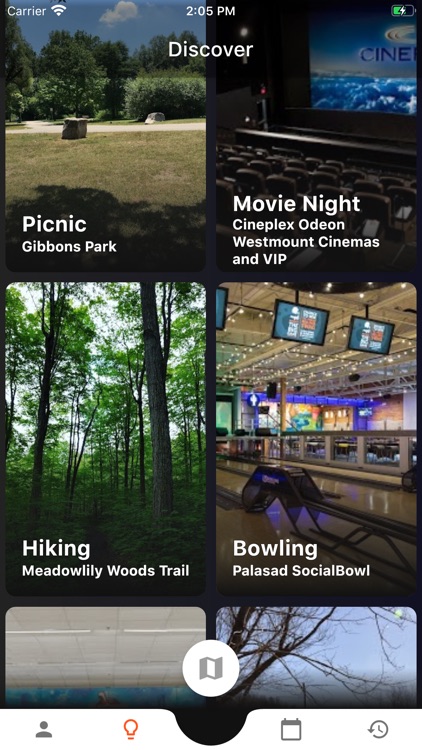This screenshot is from a smartphone, as evidenced by the status bar at the top of the screen. The time displayed is 2:05 p.m., and the battery icon on the top right shows it is less than 25% charged, yet currently being recharged, indicated by a white lightning bolt. 

The primary focus of the screen is a section labeled "Discover" located near the top-center. This section showcases four square-arranged images, each representing different activities:

1. **Top Left:** "Picnic - Gibbons Park" (caption located at the bottom left of the image).
2. **Top Right:** "Movie Night - Cineplex, Odeon, Westmount Cinemas and VIP" (caption located at the top right of the image).
3. **Bottom Left:** "Hiking - Meadow Lily Woods Trail" (caption located at the bottom left of the image).
4. **Bottom Right:** "Bowling - Palisades Social Bowl" (caption located at the bottom right of the image).

Below these images, some additional pictures are partially visible, although their captions cannot be read. This likely indicates the screen belongs to a travel or local discovery app that is highlighting various activities available in a specific area. The specific location, however, is not mentioned.

At the very bottom of the screen, there are icons for navigation. On the bottom left, there is a profile icon, and next to it, an orange location pin icon, suggesting functionalities related to user profile and location-based searches respectively.